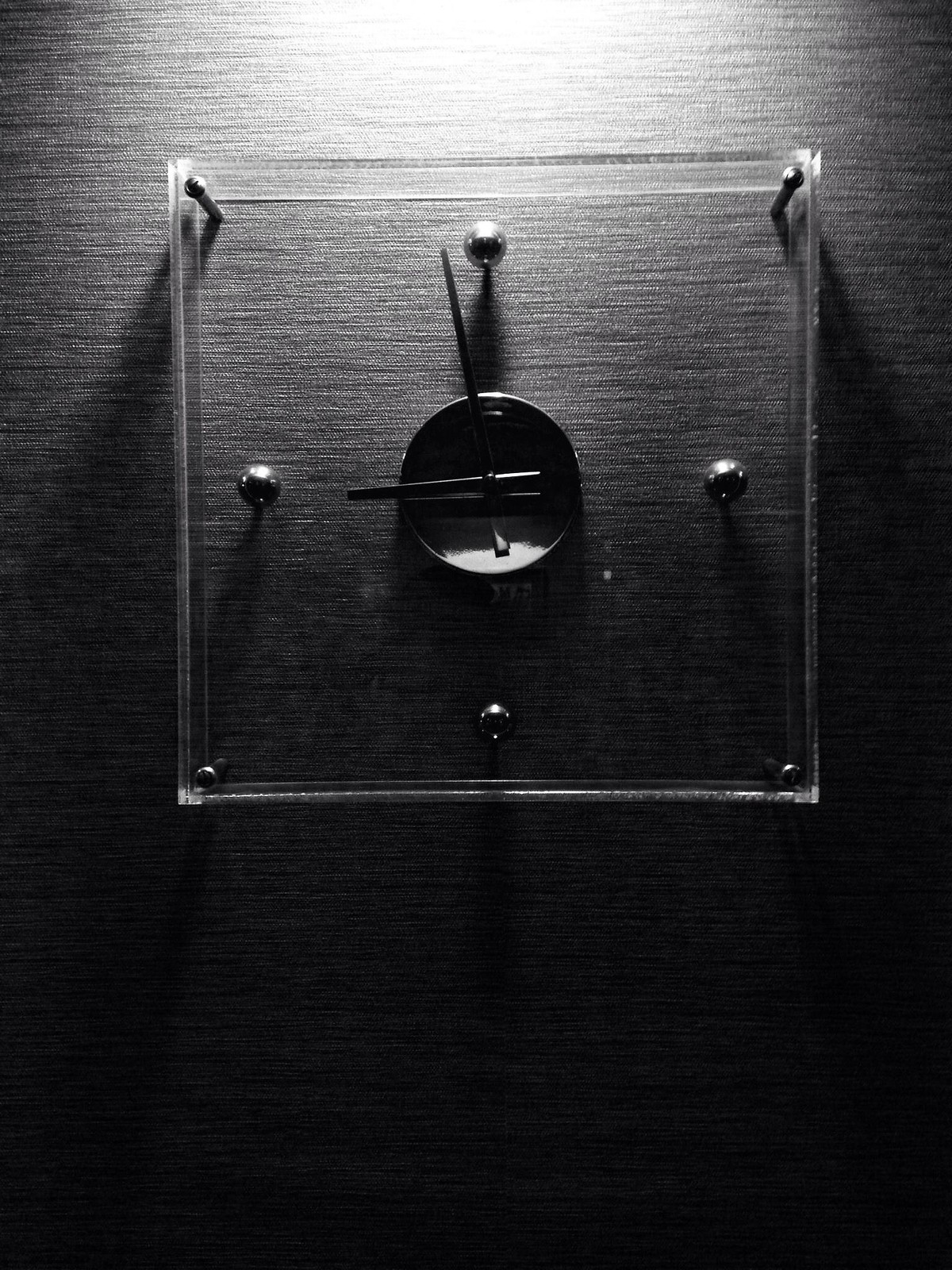This black and white photograph features a distinctive wall clock with a modern, minimalist design. The clock is encased in square plexiglass, which is held in place by four screws positioned in each corner, providing both a functional and aesthetic element. At the center of the clock is a prominent black circle from which the small, black hour and minute hands extend. The clock is showing the time as nearly 9 o'clock, precisely around 8:57 or 8:58. Surrounding the central black circle are four large, cylindrical rods placed at the 12, 3, 6, and 9 positions, indicative of the clock's key hours. The background wall is textured and predominantly gray, with a light above the clock casting a reflective glow across the surface, adding depth to the image. The entire scene, rendered in grayscale, emphasizes the sleek and elegant design of the clock against the subtly detailed backdrop.